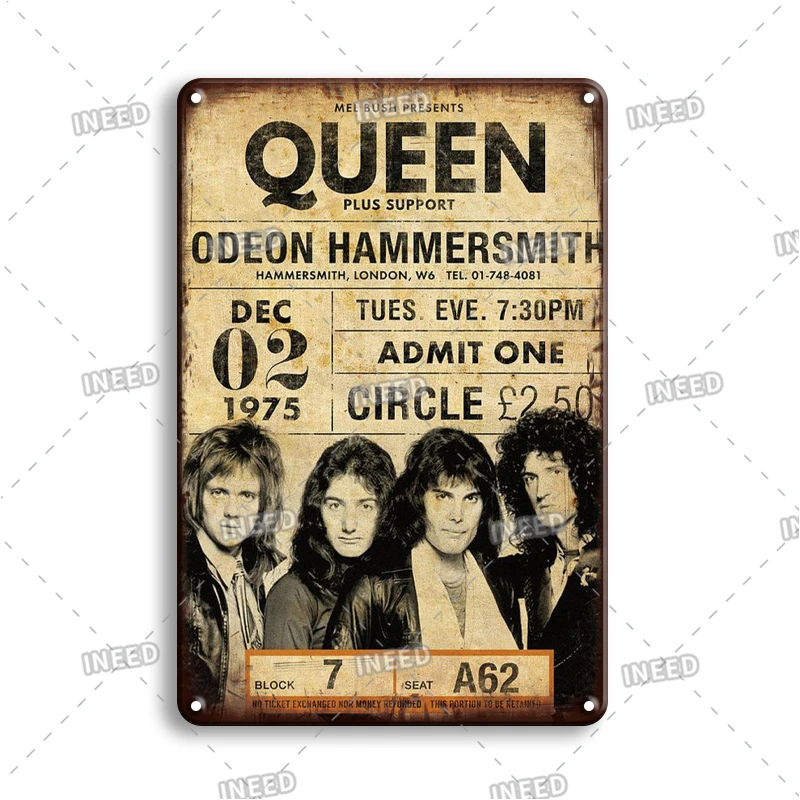The image features a white background with a repeated dotted diamond pattern that says "I need" in several spots. Overlaid on this background is a tattered, vintage-style advertisement that appears decoupaged onto a piece of wood, giving it an antiqued look. The edges of the wooden piece are darker than the center, enhancing the vintage effect. The top of the advertisement reads "Queen plus support" in black writing, followed by details of an event at the Odeon Hammersmith in Hammersmith, London, W6. The text includes a telephone number "TEL: 01-748-4081," and the date "December 02, 1975," specifying "Tuesday evening, 7.30 p.m." Further down, it states "Admit one, Circle, £2.50." Below this information is a black-and-white photograph of the four Queen band members, depicted wearing leather coats and white undershirts with long hair. The ticket's seat and aisle number "Block 7 CA 62" is also visible. The overall impression is of a nostalgic wall hanging, reminiscent of a concert ticket, possibly rendered to look like it's made of metal or wood.